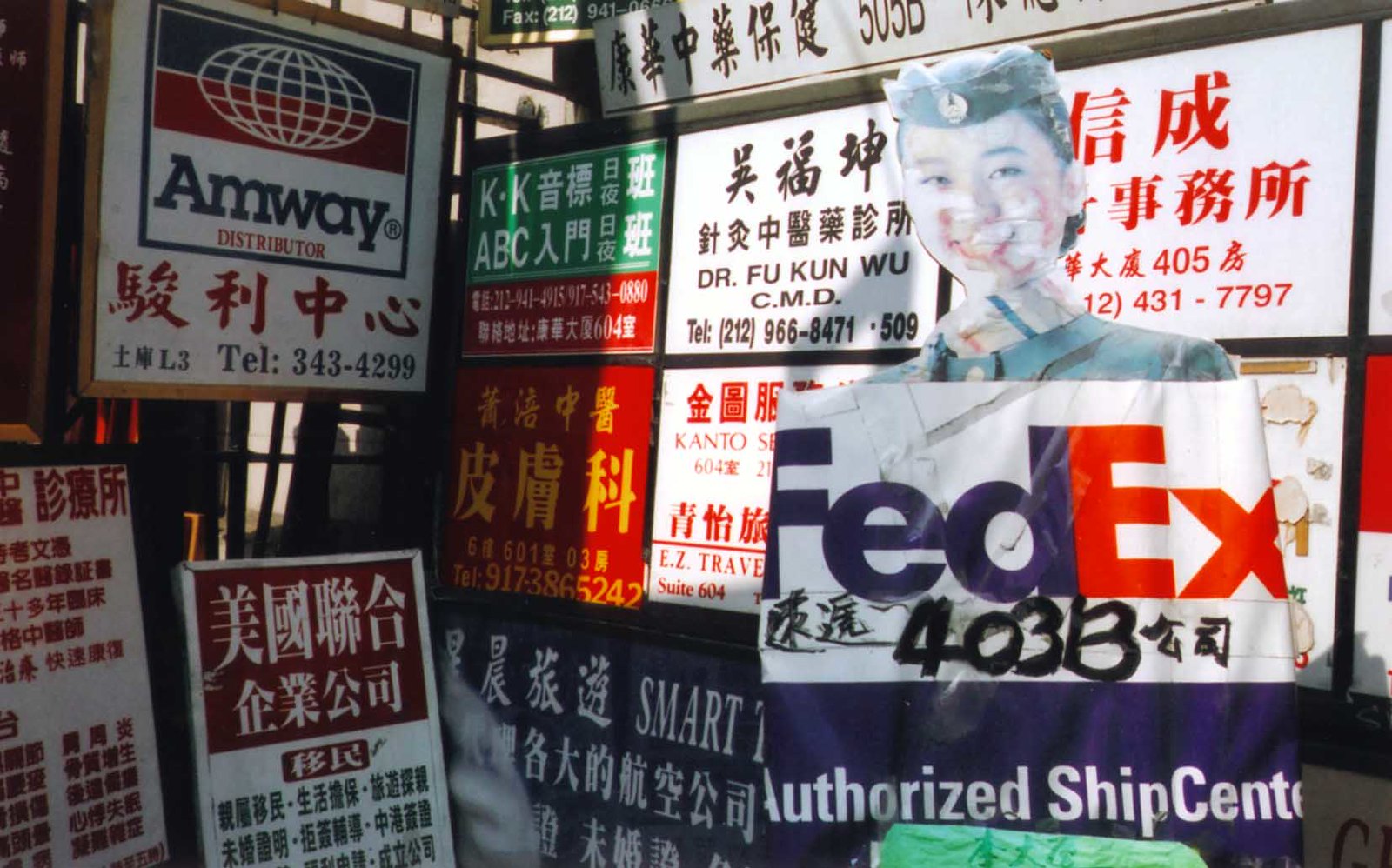The image depicts a bustling scene densely packed with Asian signage, dominated by an advertisement featuring an Asian woman, possibly adorned in a flight attendant uniform. She dons a black hat that curves around her head and a dark green uniform accentuated with a whitish scarf. She prominently holds a FedEx sign flanked by Asian text and numbers, including "403B" and "Authorized Ship Center," suggesting the location is an official shipping hub. Surrounding her sign are multiple other signs, including six smaller ones arranged in two rows behind her and a large white sign at the top filled with more Asian characters and numbers. Below the rows, a black sign is visible with Asian text and partially obscured English words with "smart" being discernible. To the left, an "Amway" sign featuring a globe icon, phone number, and more Asian text stands over two ground-level signs: one predominantly red and another with a red rectangle and white text above a section with black text. The area’s appearance evokes a market-like ambiance with numerous ads and banners, primarily consistent in Chinese text, indicating a location possibly in China.